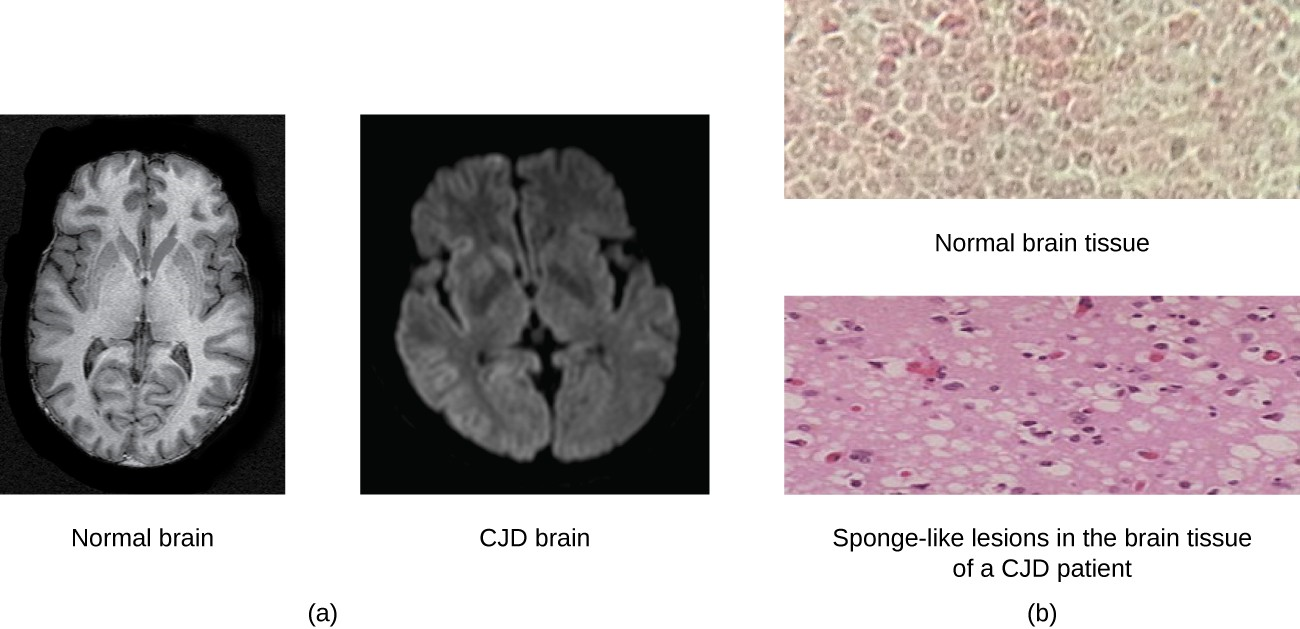The image panel showcases a set of four detailed photographs typical of a medical textbook, contrasting the structural and tissue differences between a normal brain and one affected by Creutzfeldt-Jakob Disease (CJD). 

The left side of the panel, labeled "Figure A," presents two black-and-white MRI-sliced images of the brain, both viewed from the top down against a black background. The first image, labeled "Normal Brain," depicts a brain with well-defined, symmetrical structures, primarily in white, resembling a bean-like shape. Notable areas of gray appear towards the mid-top left and right sides. Adjacent to this is the "CJD Brain," which appears asymmetrical and misshapen, with significantly reduced white areas, now predominantly gray and featuring some void spaces.

On the right side, labeled "Figure B," are two color close-ups of brain tissue under a microscope. The top image, described as "Normal Brain Tissue," exhibits a beige background with neatly arranged pink circles, indicative of healthy cellular structure. Below it, the "Sponge-Like Lesions in Brain Tissue of a CJD Patient" image stands out with a predominantly pink hue, showcasing irregular black and purple-like circles, indicative of the pathological changes caused by CJD.

This comprehensive visual comparison vividly highlights the stark differences between a healthy brain and one afflicted by CJD, both in overall structure and at the microscopic tissue level.